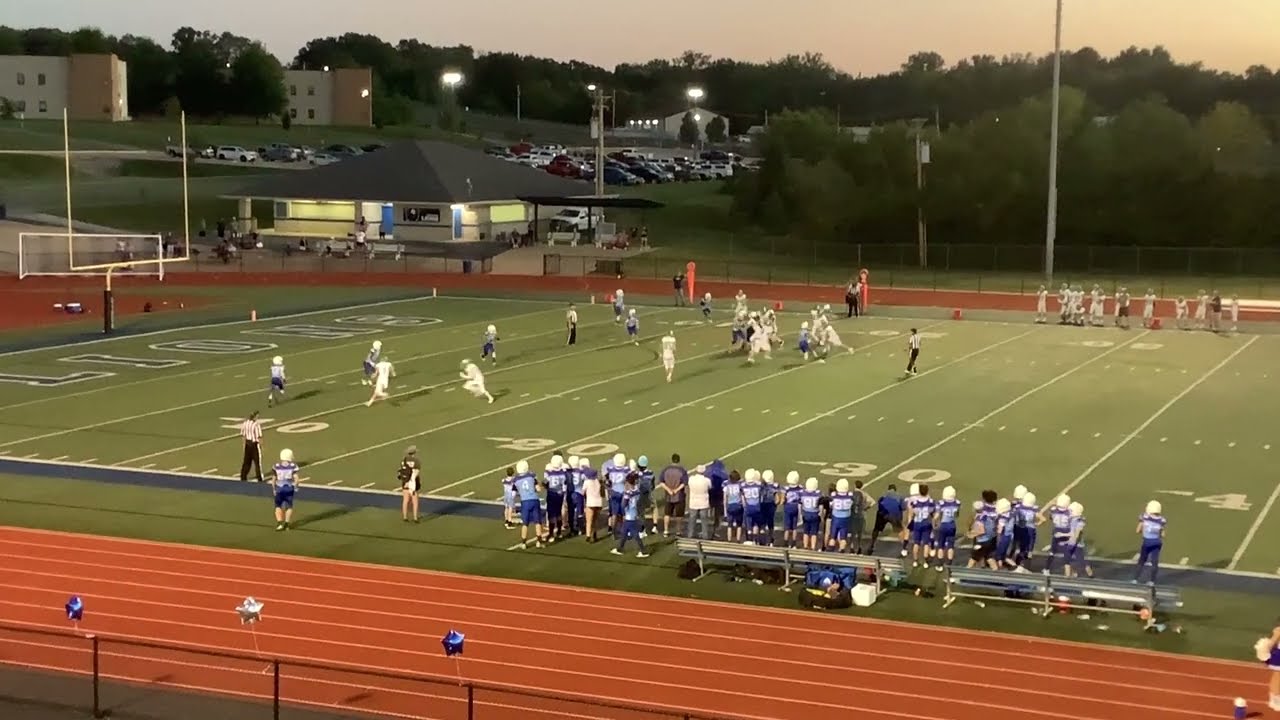This horizontal rectangular image captures the action of a high school football game, indicated by the presence of a surrounding running track and the youthful appearance of the players. The field, a lush green under stadium lighting suggesting it's nearing sunset, hosts teams in white and blue uniforms. The game is in progress, with the offense in white advancing around the 15-yard line towards the far goal posts, their end zone partly obscured but marked by visible numeric boundary lines such as 10, 20, and 30.

In the foreground, the majority of the blue team is gathered on the sideline, anxiously observing their teammates defending the field. A reddish-brown running track with multiple lanes encircles the field, and tied to the fence on the bottom left are three balloons, adding a festive touch to the scene. Beyond the track, a fence separates the field from other infrastructure, which includes a visible parking lot, a lighted area likely belonging to the school, and green trees in the distance. The image appears slightly pixelated, hinting it might be a screenshot from a video rather than a conventional photograph.